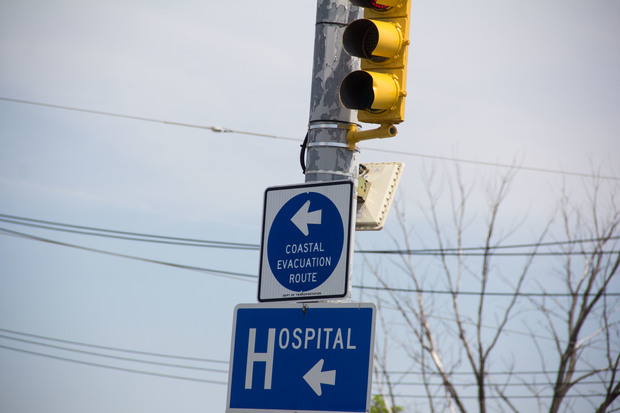In the photograph, a centrally positioned silver pole serves as the focal point against a backdrop of gray, cloudy skies. Mounted at the top of this pole is a yellow traffic light, consisting of red, yellow, and green signals. Below the traffic light, there's a blue and white sign indicating the "Coastal Evacuation Route," with a white arrow pointing to the left. Beneath this sign, another blue and white sign directs towards the "Hospital," also with an arrow pointing to the left. Surrounding the pole are power lines and communication lines that stretch horizontally, with trees visible behind them. The scene is tranquil, devoid of people, and the overcast, yet bright, day highlights the detailed signage and infrastructure, suggesting an urban or suburban setting.